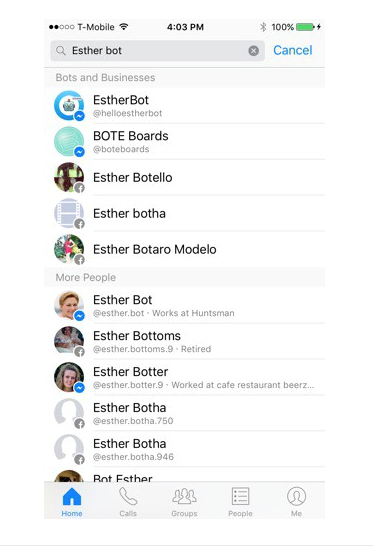A screenshot from a smartphone reveals a search result page for "Esther bot". At the top, under the category "Bots and Businesses," the search result for "Esther bot Helios" is displayed. Below it, various search results for "Esther bot" and related names appear, including "Boat a boards," "Esther Bortello," "Esther Bordeaux Mordella," and many more variations featuring the name "Esther" followed by different suffixes.

The screen further down shows a "More people" section, listing names such as "Esther Bottoms," "Esther A Bot Her," and "Bot Esther Bear," along with profile pictures of these individuals.

At the bottom of the screenshot, a navigation menu is visible, consisting of icons for "Home," "Calls," "Groups," "People," and "Me," indicating different sections of the mobile application.